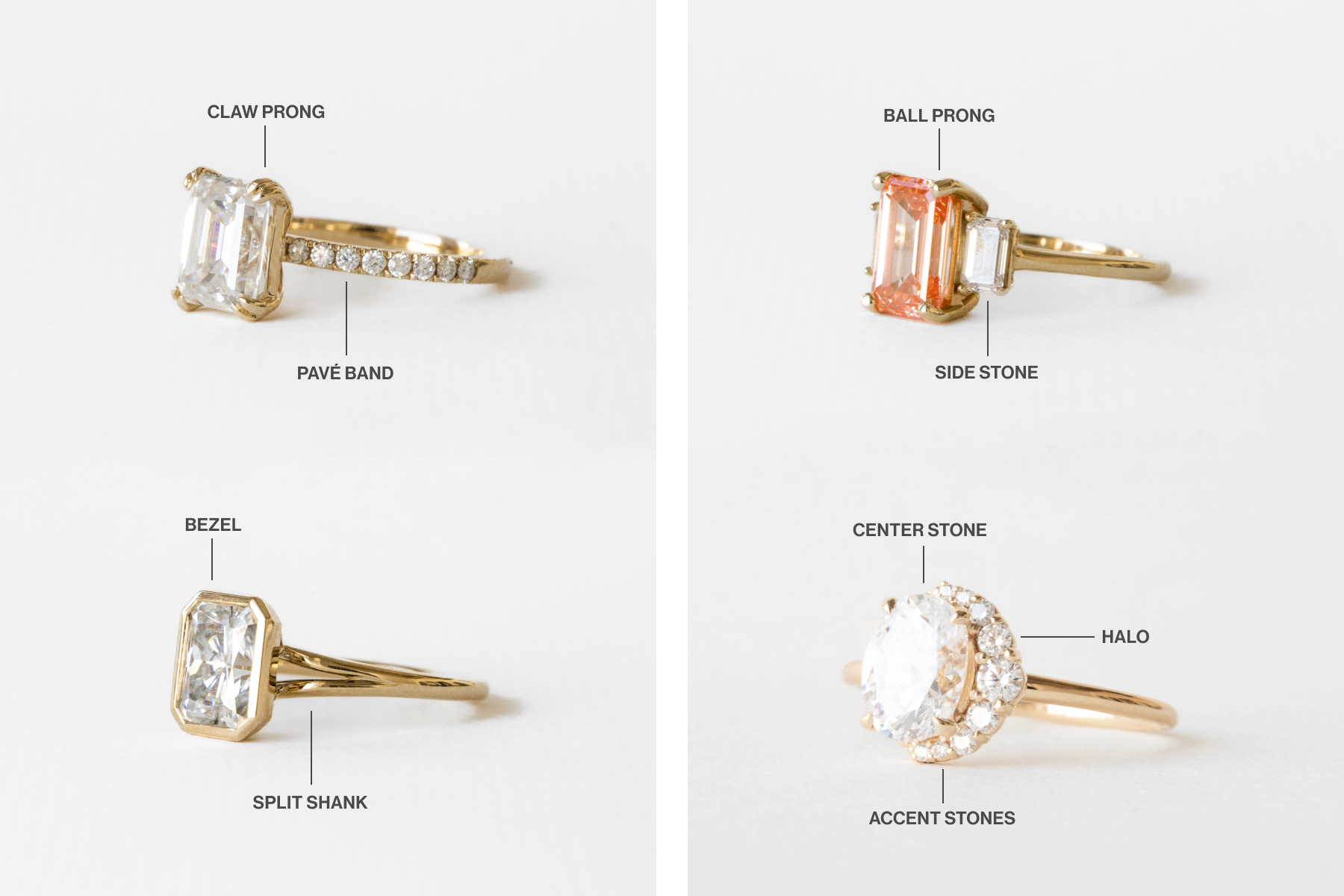The image depicts a set of four distinct engagement rings arranged in two columns against a light gray background. Each ring features detailed labels highlighting its unique design elements. 

- The top left ring showcases a large, square-shaped white diamond flanked by smaller diamonds along its band, denoted as "claw prong" and "pave band." It is set in gold.
  
- The ring on the top right displays a pinkish, reddish transparent stone accompanied by a smaller white gem on a standard gold band. It includes the terms "ball prong" and "side stone."

- The bottom left ring has a rectangular diamond with angled corners on a thin, plain gold band. It is described as having a "bezel" setting with a "split shank."

- The bottom right ring is the most elaborate, featuring a prominent central white gem encircled by smaller diamonds. The band and halo are also adorned with additional diamonds, labeled as "center stone," "halo," and "accent stones."

The overall image serves as a detailed guide to various engagement ring styles, perfect for anyone looking to understand different ring settings and designs.